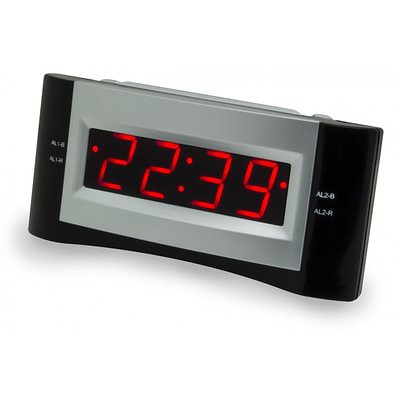The photo is set against a white background and features a digital alarm clock positioned at an angle, extending from the top left-hand corner to the bottom right-hand corner. The clock itself is rectangular but has a slight indentation at the bottom, tapering towards the center. Surrounding the display is a black border, within which sits a gray rectangle. Inside this gray rectangle is a black display area that showcases the current time in red digital numbers: 22:39, corresponding to 10:39 p.m. The numbers are framed by a pattern of dots, including a colon between the hours and minutes, two dots above each other, and an additional dot to the right. On either side of the gray display, white text is visible, though its focus is somewhat soft, with some letters appearing to read ALZ-B and AL2-R. The perimeter of the clock's display is silver, contrasting against the predominantly black and gray design, possibly indicating it is made of metal or hard plastic.